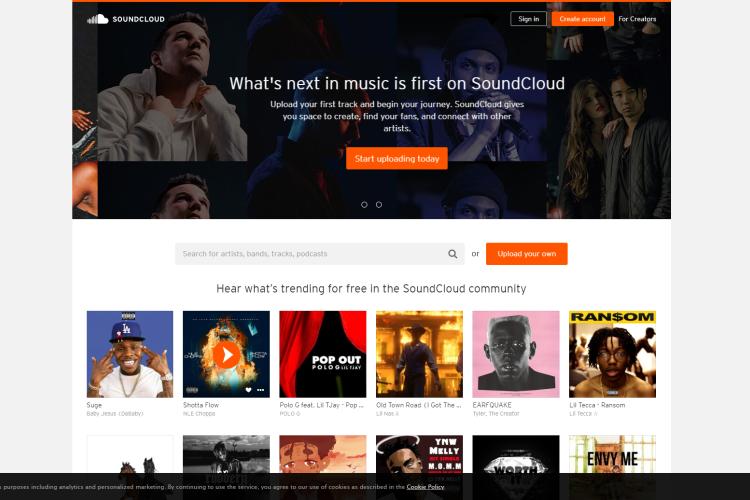The image is a screenshot of a website that is 30% wider than it is tall. The overall color scheme is predominantly dark, featuring a black background with subtle blue hues. The banner at the top is predominantly black with accented blue tones. On the upper left side of the banner, there is a white "SoundCloud" logo consisting of a cloud icon followed by the word "SoundCloud" in all capital letters. 

On the upper right side of the banner are two buttons: a black "Sign In" button outlined in white with white text, and an orange "Create Account" button with white text. To the right of these buttons is the phrase "For Creators," written in white, without any background.

The central background of the webpage is composed of various profile shots. Overlaid in the center is bold, white text that reads, "What's next in music is first on SoundCloud." Below this central text are three lines of smaller white text. Completing this section is an orange button with white text that says, "Start uploading today."

Below this, there is a search bar followed by a grid displaying what appear to be album covers or artist profiles. The grid consists of six columns and two rows of album-like images.